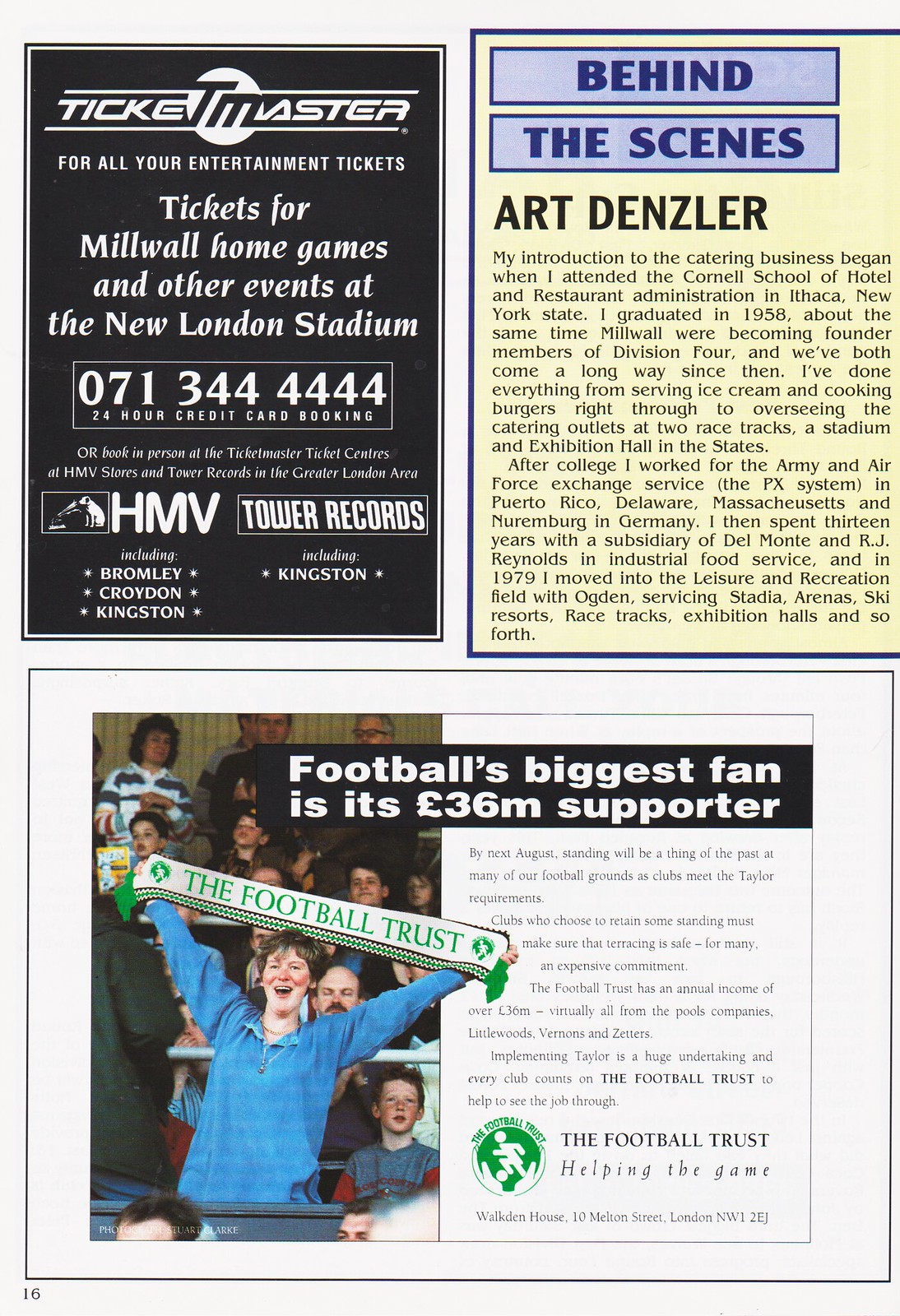This magazine page features a variety of advertisements vividly capturing different aspects of entertainment and sports. At the top left, a prominent black-and-white advert for Ticketmaster stands out with the bold text "Ticketmaster for all your entertainment tickets." It specifically highlights tickets for Millwall home games and other events at the new London Stadium, with a 24-hour credit card booking number: 071-344-4444. Below this, the text reads "HMV and Tower Records," accompanied by a nostalgic image of a dog with a gramophone. 

To the right, another eye-catching ad bordered in yellow and blue promotes an exhibit hall introduction titled "Behind the Scenes" featuring Art Denzler.

Dominating the lower half of the page is a vibrant image of a woman passionately holding up a banner for "The Football Trust" with the slogan "Football's biggest fan is its 36 million supporters." She stands proudly among a crowd, donning a blue shirt and a gleaming smile, symbolizing the fervent support of football fans everywhere. The ad also showcases the green logo of The Football Trust.

Overall, this page is a lively collage that encapsulates the essence of entertainment ticketing, exhibition hall previews, and the passionate fan base of football.